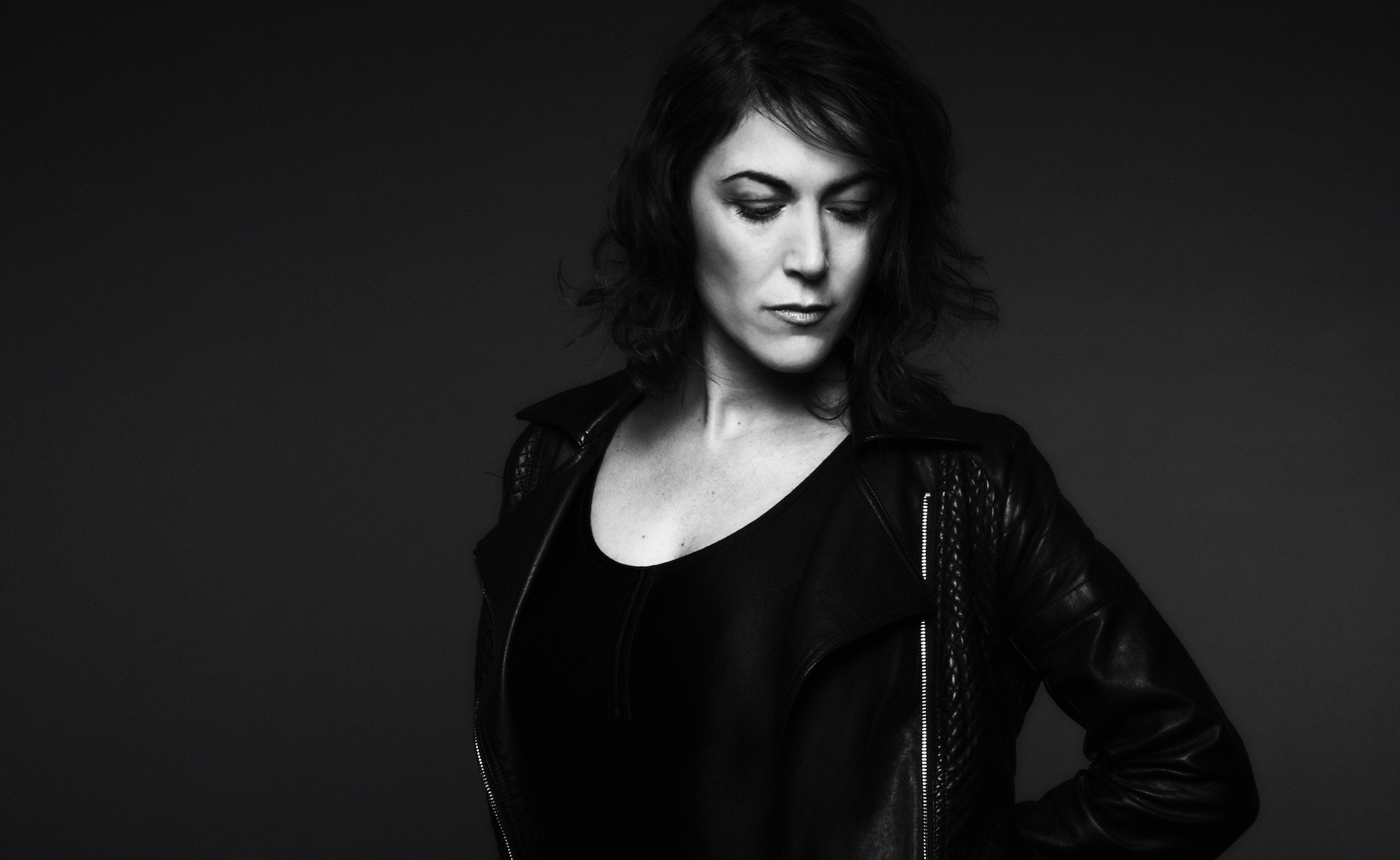In this striking black and white photograph, a woman with slightly wavy black hair, which reaches down to her shoulders, stands against a dark gray background. She is dressed in a stylish black leather jacket, identifiable by its metal zipper, worn over a black scoop neck top. The woman appears to be in her early 40s. She gazes downward toward the bottom right corner of the image, giving her face a neutral yet introspective expression. Her dark eyebrows and long, mascara-coated eyelashes stand out, emphasizing her closed or nearly shut eyes. One of her arms is bent with an elbow slightly out, suggesting her hand is either on her hip or behind her back, while the other hand is situated behind her. Her hair has a slight wave, adding a touch of volume as it poofs out subtly at the sides, completing the chic and composed look captured in the image.